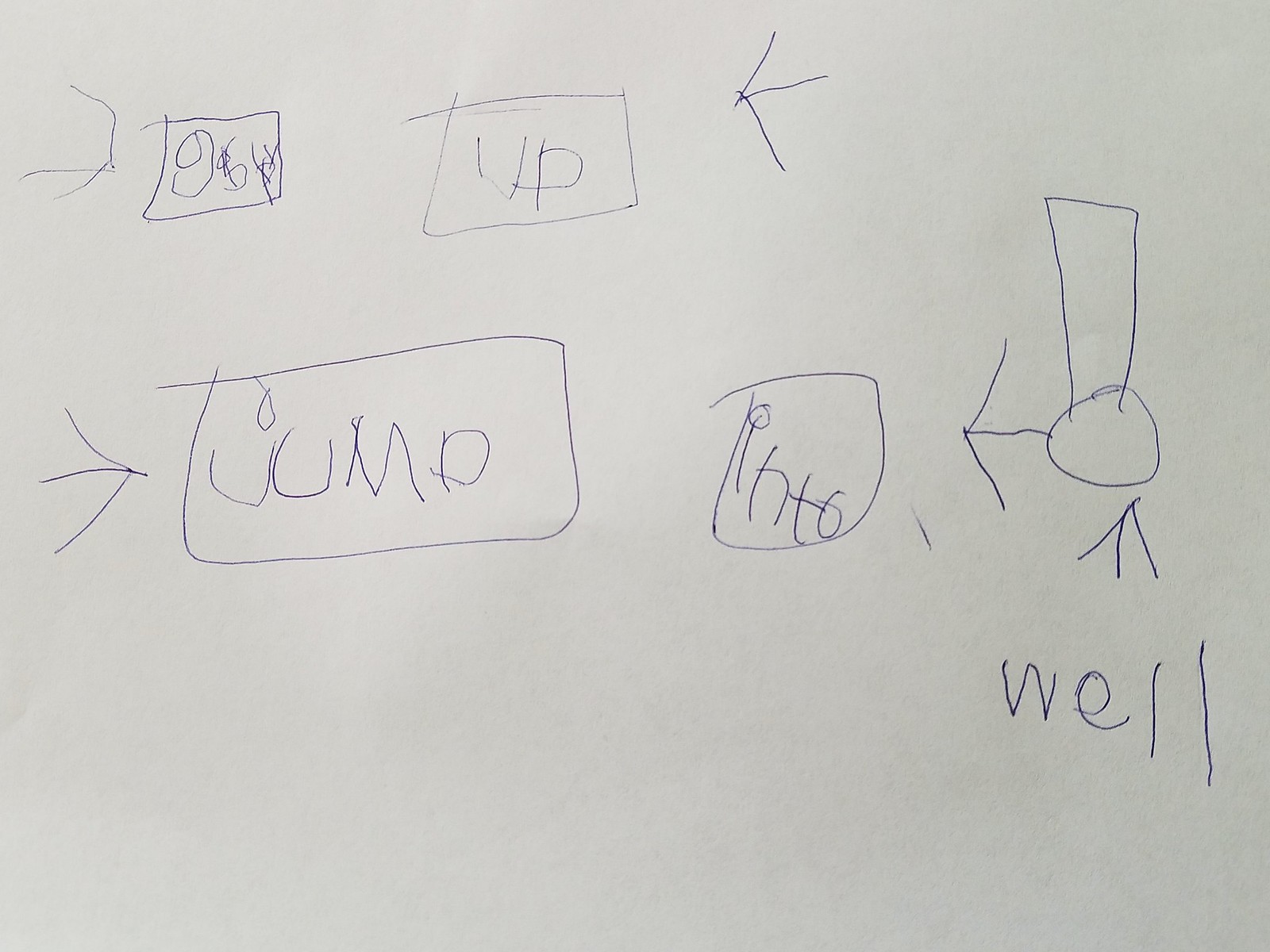In this image, there is a white piece of paper featuring an array of drawings made with a blue ink pen. At the top of the paper, two small, sloppily drawn squares are positioned side by side. The first square contains unclear, scribbled letters that appear to be "G," "S," and "Y," though some letters are overwritten and difficult to decipher. An arrow to the left of this square points right towards it. The second square has "U," "P" written inside it, and an arrow on the right side of this square points left towards the text "UP."

Below these two squares is a larger rectangle that stretches horizontally, with the word "JUMP" written inside it. An arrow to the left of this rectangle points right towards the word "JUMP." To the right of the large rectangle is another smaller square box containing the word "INTO," written in capital letters and also sloppily drawn.

To the right of the "INTO" box, there is a complex shape consisting of a circle with a vertical rectangle emerging from its top. An arrow extends from this circle-rectangle shape, pointing left towards the "INTO" box. Below this shape, the word "WELL" is written ("W-E-L-L"), and there is an arrow above the word "WELL" pointing upwards towards the circular part of the circle-rectangle figure.